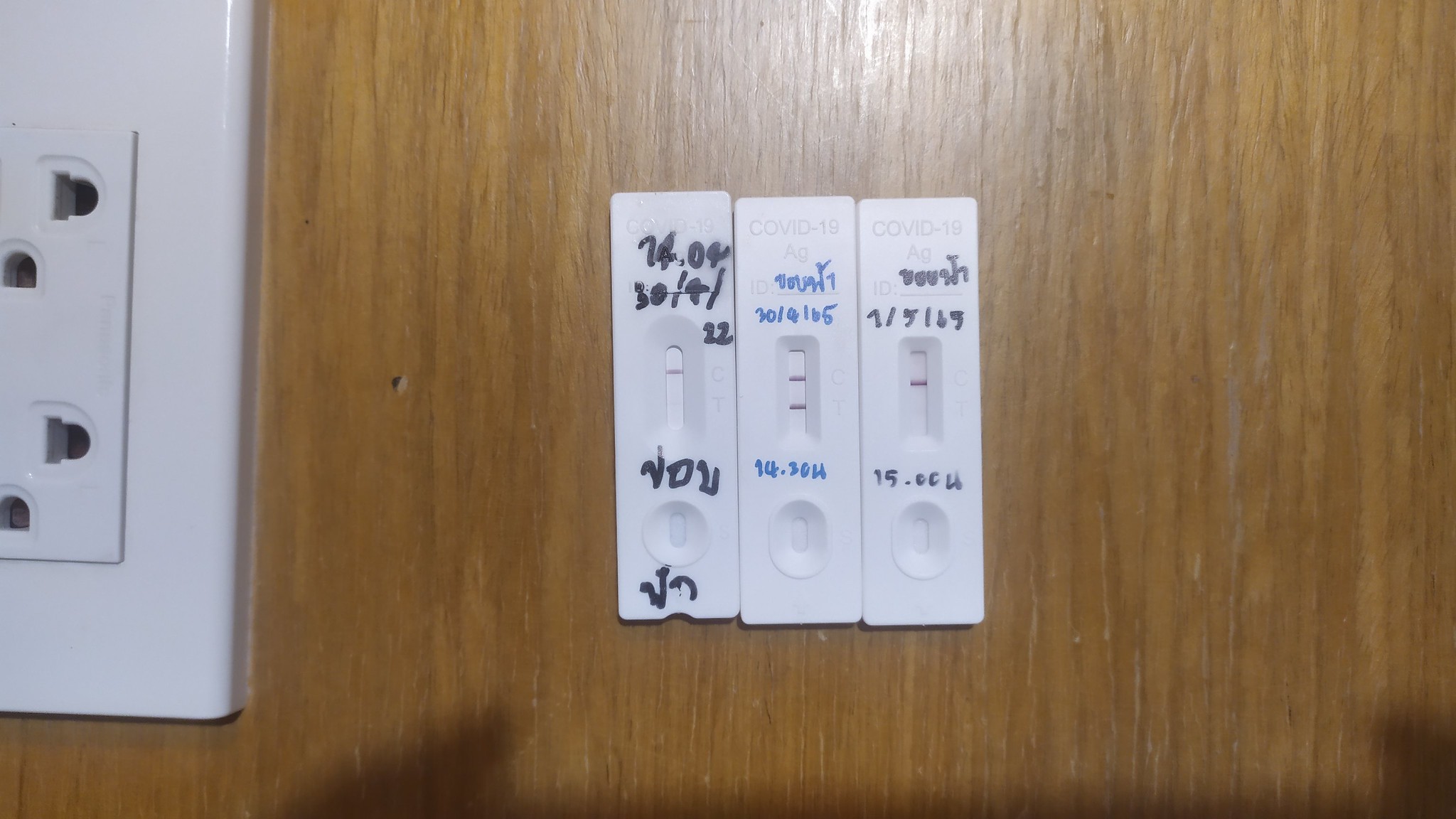The image features three COVID-19 test devices prominently labeled with "COVID-19" at the top. Below this label, each device displays “AgID:” followed by a line. The tests are housed in white rectangular casings, which appear to be made of plastic or a similar material. 

The three devices are slightly varied in design. The leftmost test has a unique feature—a rounded notch at the bottom center of its casing. The lower section of this device includes an indented oval and a surrounding circular shape.

The two tests on the right share an identical design, featuring a vertical oval inset in their lower sections, surrounded by a wider oval shape. 

All three devices display handwritten annotations using different colors of Sharpie: black on the leftmost test, blue in the middle, and black on the rightmost one. 

The tests appear to be mounted or placed against a wall that has a varnished finish, indicating a potential wooden surface. To the left of the tests, part of an electrical outlet is visible, including its inner components and the outer border, which are likely made of plastic or another similar material.